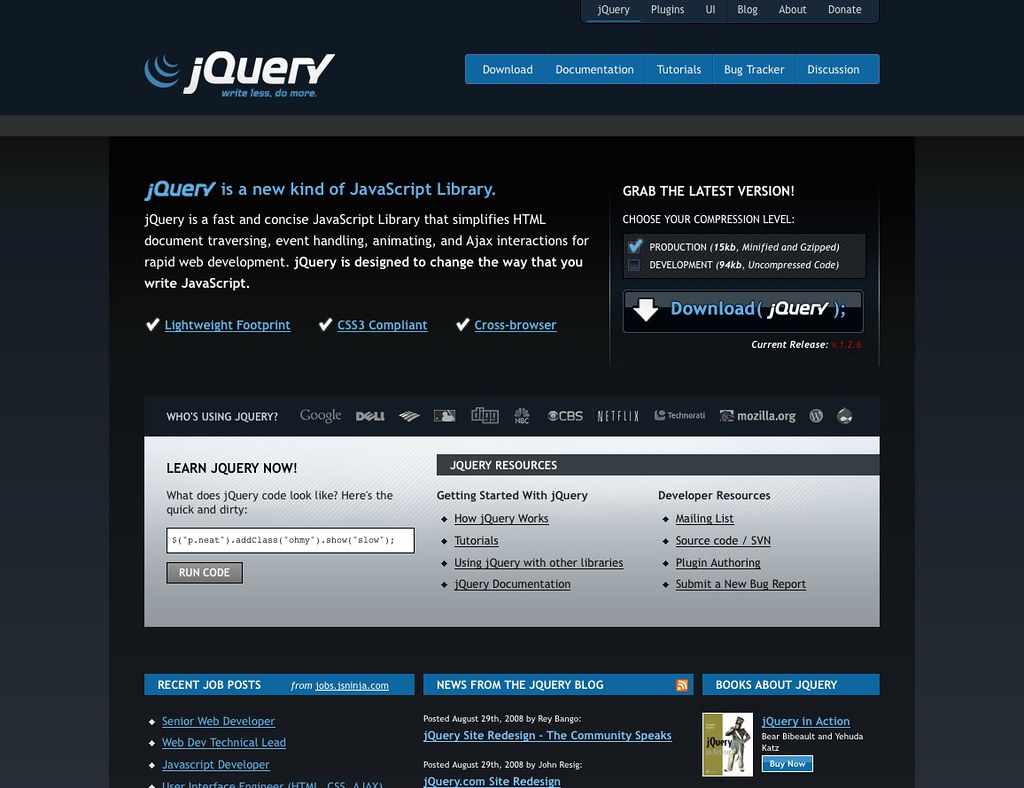The image depicts a dark-themed website with a focus on the jQuery JavaScript library. In the top left corner, the name "jQuery" is prominently displayed in white text, accompanied by its logo—three light blue boomerang-like shapes. Directly beneath the jQuery name is the slogan, "Write Less, Do More," also in light blue.

To the right of the logo and slogan, a series of categories are listed in white text: "Download," "Documentation," "Tutorials," "Bug Tracker," and "Discussion." Above these, more site navigation options are presented at the top right corner, including "jQuery," "Plugins," "UI," "Blog," "About Us," and "Donate."

Separating the main content from the header is a horizontal blue bar. Centered towards the upper-left section of the image, the headline reads, "jQuery is a new kind of JavaScript library," followed by a descriptive paragraph. It states that "jQuery is a fast and concise JavaScript library that simplifies HTML document traversing, event handling, animating, and AJAX interactions for rapid web development. jQuery is designed to change the way that you write JavaScript."

Further down, three key features of jQuery are highlighted with a white check mark to the left of each: "Lightweight Footprint," "CSS3 Compliant," and "Cross-Browser Compatibility."